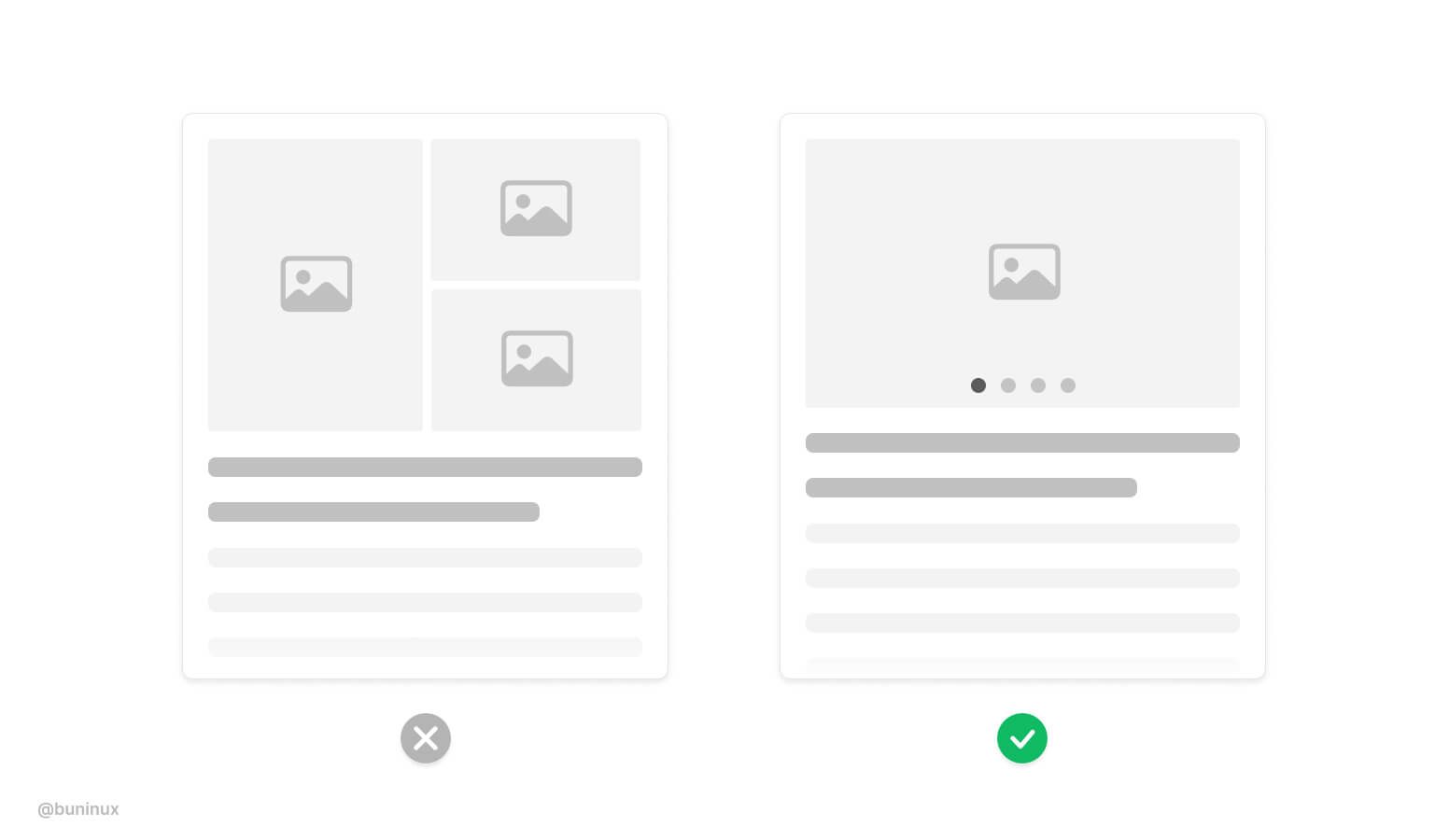The picture displays two grey-toned design mockups, each showcasing distinct layout templates for content. 

In the first mockup, there are three image placeholders comprising one large and two smaller images, the combined size of which matches the large image. Beneath these placeholders is a designated area for text, currently appearing as a placeholder. At the very bottom sits an 'X' symbol within a grey circle.

The second mockup features a slightly different layout. It includes a single large placeholder for an image, occupying the same overall space as the three images in the first layout. Below this placeholder, there is also a similar text area. Notably, this image has a small navigation indicator beside it, allowing up to four images to be cycled through, indicating it is set to show 'image 1 of 4'. At the bottom of this mockup is a green tick mark, the only element of color present in either image.